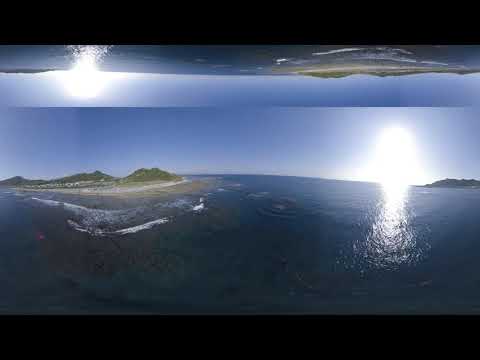This image portrays a panoramic outdoor scene taken from the perspective of someone in the ocean during midday. The composition features a solid black border running across the top and bottom. The vivid scenery is split by a body of dark blue water occupying the entire lower half, reflecting a bright sun positioned in the upper right corner. To the left of the image, there is a prominent island adorned with green hills, dense shrubs or trees, and a sandy tan beach. The waves crash against this island, creating a dynamic interplay with the water. The sky is mostly clear except for the glowing presence of the sun. Further in the distance, another island with similar greenery is faintly visible on the right side. The image's top portion seems to be a flipped and cropped reflection of the main scene, showing the sun and island mirrored on opposite sides. Colors in the picture range from black and dark blue to shades of green, tan, and light blue, contributing to a serene and picturesque panorama.